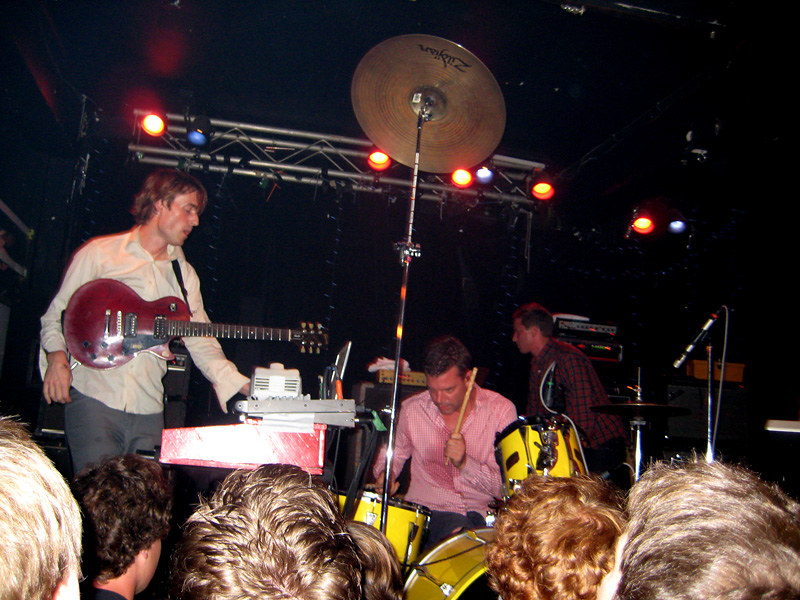A lively band performance captured in vibrant detail: In the foreground, a passionate guitarist with their instrument slung high on their chest strums energetically. The drummer, drenched in sweat, pounds on a set of striking yellow drums, dressed in a bold pink button-down shirt. In the background, a figure in a flannel shirt adds to the scene's energetic ambiance. The tops of five heads with unruly hair peek into the frame, emphasizing the crowd's enthusiasm. Dominating the front is a towering cymbal, accompanied by vivid orange and blue stage lights, illuminating the dynamic and electric atmosphere of the concert.